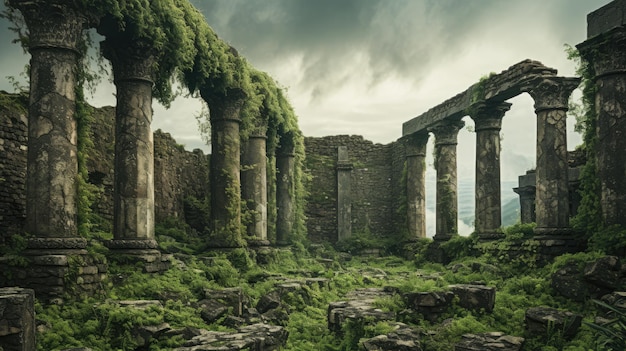The image depicts an AI-generated artwork of an abandoned, ancient structure, reminiscent of Roman or Greek ruins, situated in an outdoor setting. Dominated by a pair of lengthy, statue-like buildings, each featuring a series of four or five tall pillars, the scene exudes an air of desolation and decay. These pillars, partly covered in moss and vines, are connected overhead by long cement beams, suggesting they once supported walls or ceilings now long gone. Scattered among the tall, overgrown green bushes and rocks on the ground lies a mix of grass, stone debris, and dilapidated stonework, further illustrating the state of ruin. Adding to the eerie ambiance is a background of a massive stone or brick building running along the left side, while the cloudy, dark sky above ranges from ominous black to murky white-gray, casting a gloomy atmosphere over the entire scene.